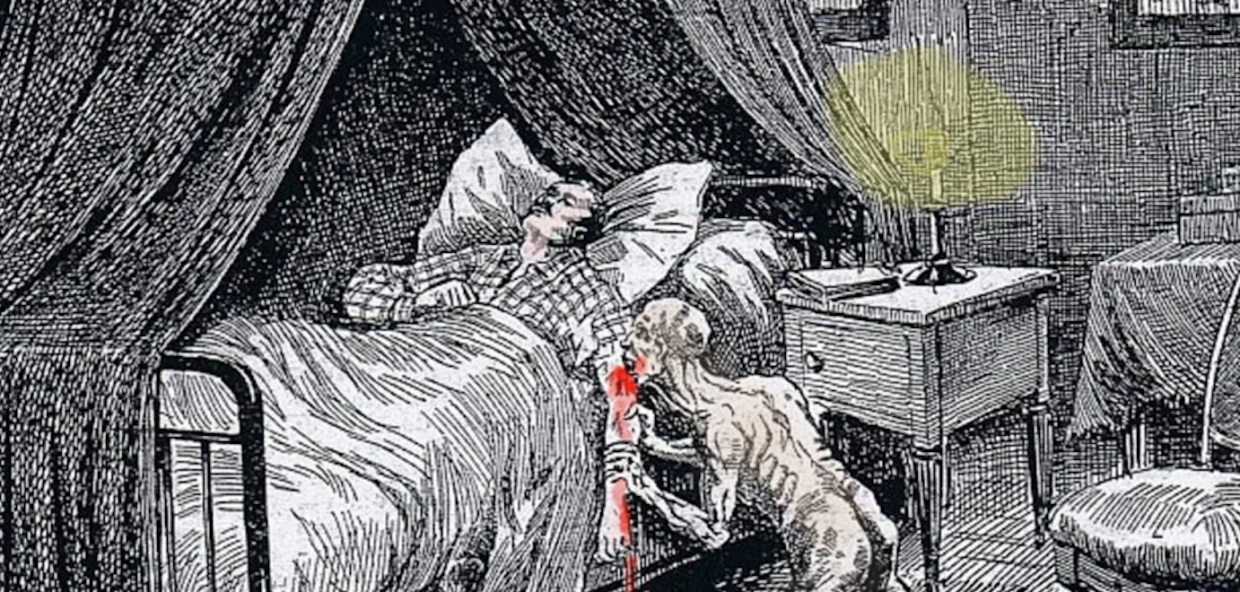This is a detailed pen and paper drawing featuring Nosferatu, a scrawny and naked vampire, drinking the blood of a man from his arm. The scene is predominantly rendered in black, white, and gray, but the blood dripping from the man's arm and the flame of a lit candle provide stark splashes of red and yellow. The man, wearing a black and white checkered shirt, lies in an iron post bed with his head on two big fluffy white pillows and a white blanket covering him up to his chest. His arm dangles over the side of the bed, blood dripping onto the floor beneath. The bed is surrounded by tied-back curtains. Nosferatu, appearing malnourished with visible ribs and spots of scar tissue on his body, kneels beside the bed, feasting on the man's arm. The nightstand beside the bed holds a lit candle and a book, casting a yellow light. In the background, there's another table with a tablecloth, a chair, and two indistinct picture frames on the wall. The intricate line work and limited color palette create a haunting, eerie atmosphere.